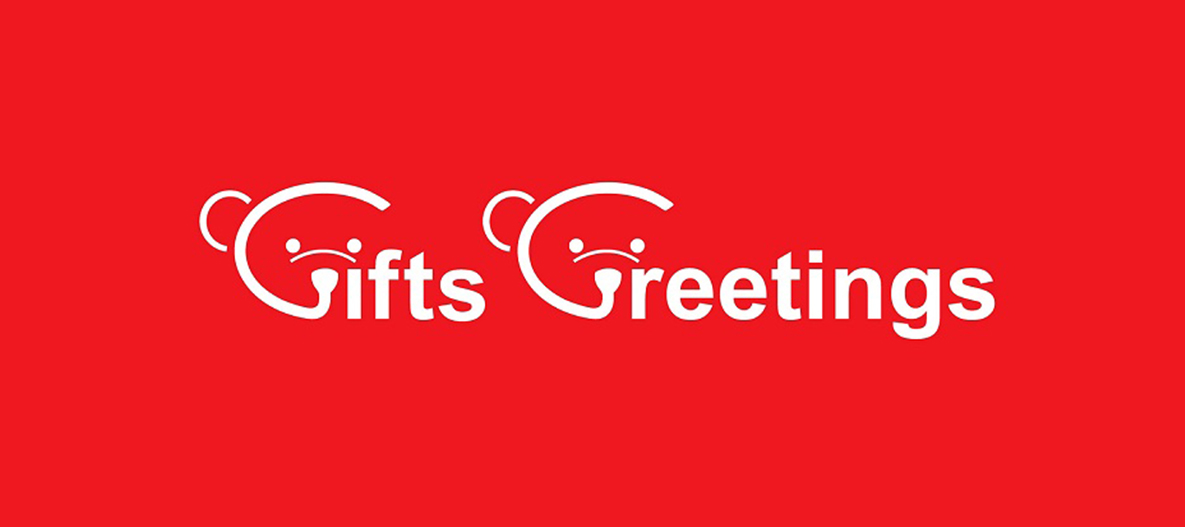The image appears to be of a festive card, characterized by a bright, Christmas-red background. The text "Gifts and Greetings" is prominently displayed in white, with each 'G' capitalized. The 'G' is creatively designed to resemble a teddy bear, complete with a small ear on the upper-right exterior of the letter. Additionally, the inside top curve of the 'G' features a tiny, sloping nose that resembles half a parenthesis, along with two small dots positioned above as eyes, giving the 'G' an adorable and endearing appearance.